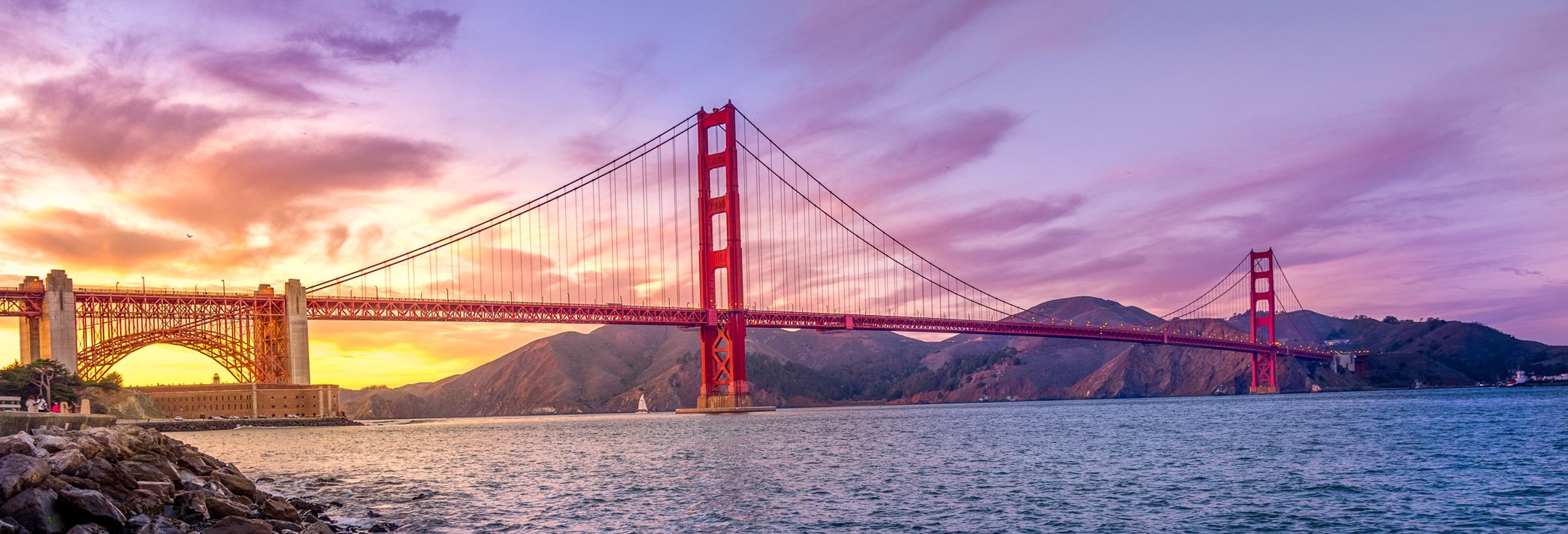This panoramic photograph of San Francisco's Golden Gate Bridge captures the iconic structure extending across the entire image. The red bridge, with its arching supports, stands out against a vividly colorful sky adorned with hues of purple, pink, orange, and yellow, suggesting it was taken during either sunrise or sunset. In the foreground on the left, a cluster of brown rocks emerges from the blue water, providing a natural contrast to the man-made splendor. Distant green tree-covered mountain ranges further enrich the landscape. In the far distance, a brown building is visible. The scene is not only a stunning depiction of architecture but also a magnificent portrayal of the city’s natural beauty.